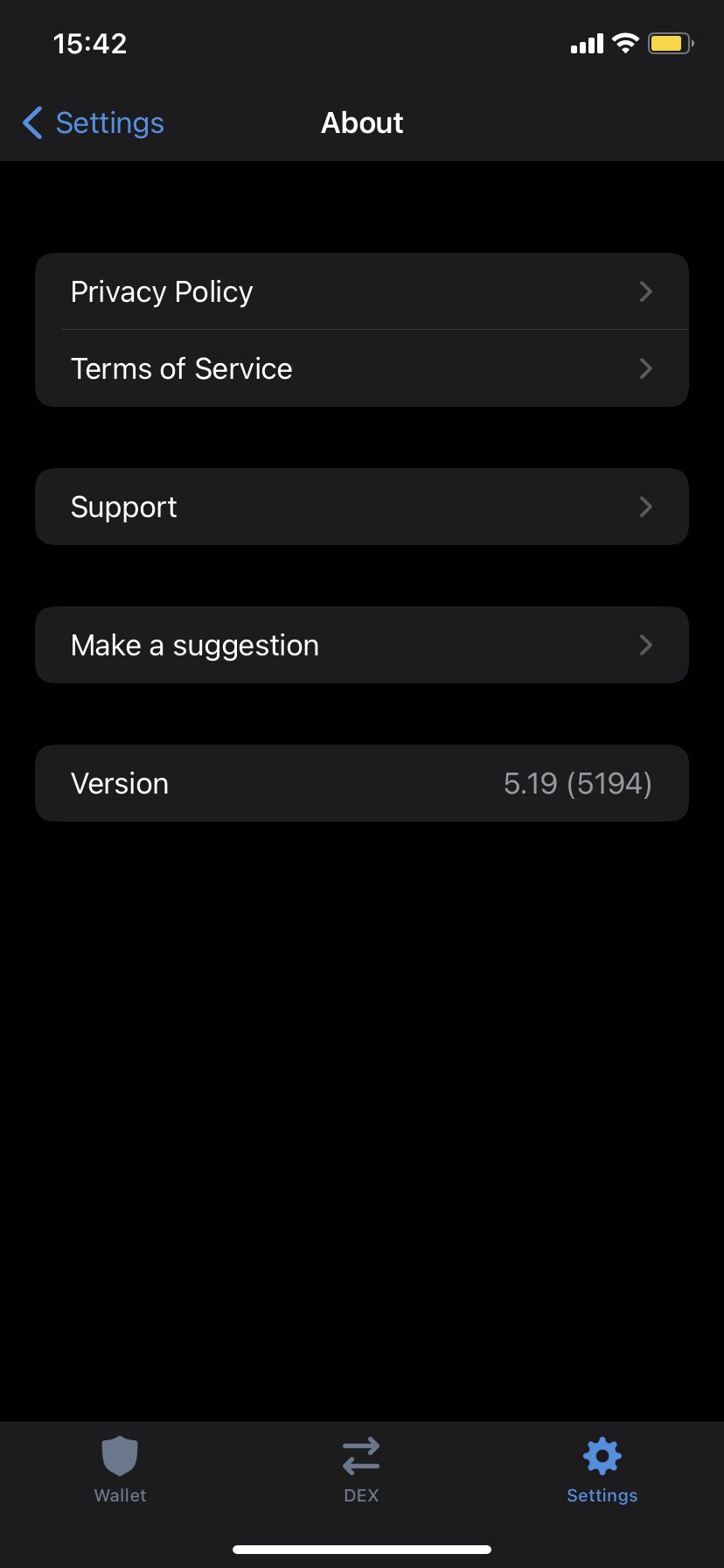This black-themed image appears to be a screenshot taken from a mobile phone's screen, likely showing a settings menu. In the top-left corner, the time is displayed as `15:42`, indicating the moment the screenshot was captured. To the right of the time, there are four white bars signifying strong network signal strength, alongside a WiFi icon resembling a fan. Beside these icons is a yellow, rectangular-shaped battery icon indicating the current battery status.

The middle section of the image is dominated by the word "Settings" written in blue. Directly below this, at the center, is the word "About." The image categorizes various sections:
- "Privacy Policy" in white text
- "Terms of Service" in white text directly beneath it
- "Support" in white text
- "Make a Suggestion" in white text
- "Version" in white text followed by the numbers `5.19 (5194)` aligned to the far right.

At the bottom of the image, there is a gray-shaded area featuring three options with icons:
1. "Wallet" accompanied by a corresponding icon
2. "Dex" (D-E-X) indicated with an icon that includes arrows pointing left and right
3. A pinwheel icon next to the word "Settings."

This screenshot provides a comprehensive snapshot of the phone’s settings page, highlighting different sections available for user preferences and information.